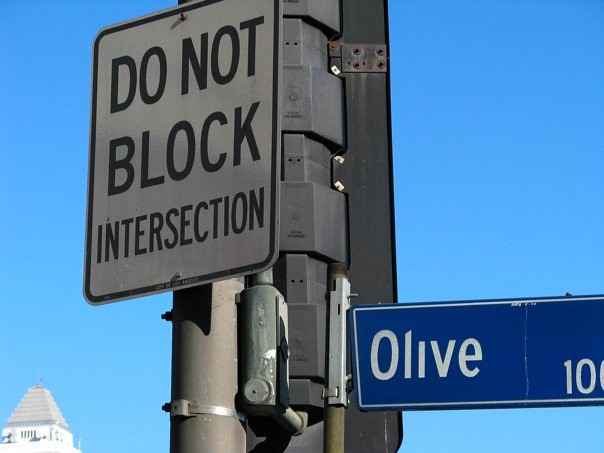This is a bright and clear close-up photograph taken outdoors, looking slightly upward at a street pole holding multiple signs against a vibrant blue sky. Dominating the foreground, a large gray pole supports two main signs. On the left, a gray sign with a black outline and black lettering reads "DO NOT BLOCK INTERSECTION." On the right, a blue sign with white lettering states "Olive 100," though the final zero is partially cut off. This sign appears to have a crack running down its middle. In the background, to the bottom left, stands the top portion of a white high-rise building with a layered, gray, triangular-shaped roof that comes to a point. The back of another sign, possibly a traffic signal due to its bulky appearance, is also visible but not legible. The scene is clean and minimalistic, focusing on the signs and the clear blue sky without any clouds.